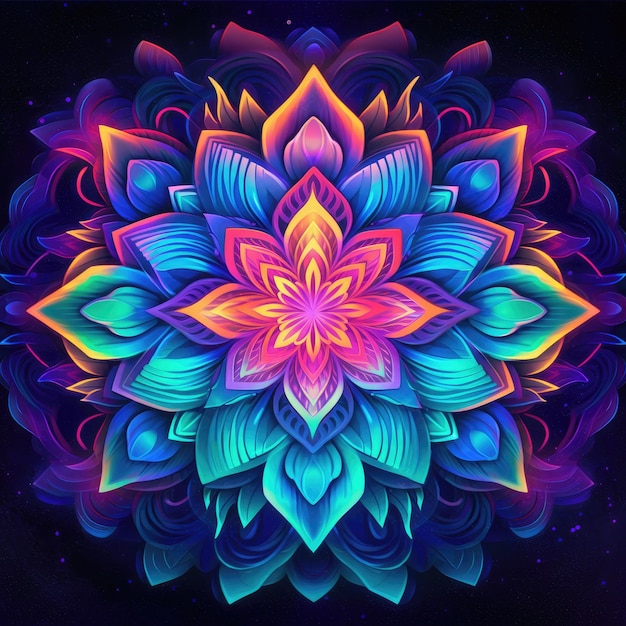The image is a stylized digital illustration of an expanding, multi-petaled flower. At its center is a vibrant, eight-sided flower that starts with a striking combination of purple and yellow. Each successive layer of petals grows larger, transitioning through a spectrum of vivid colors—yellow shifting to orange, purple blending into blue, and finally blue-green petals tinted with bright orange tips that give a flame-like appearance. The intricate petals are detailed with lines and shell-shaped patterns. This flower's layers appear to expand infinitely against a black backdrop accented by a few blue-purple dots. The outermost petals culminate in large, star-like shapes, bordered in yellow, with blue interiors and purple swirls of paint creating a ribbon-like effect. The overall composition evokes the intricate design of a mandala, but with a uniquely floral, fantastical twist.